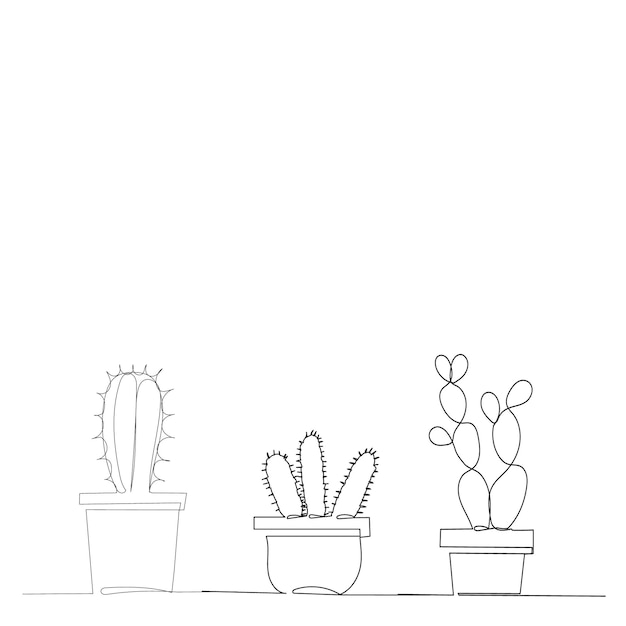The image showcases a minimalist yet striking line drawing, likely created with pencil or pen, depicting three distinct types of cacti. Each plant is potted in traditionally shaped containers and drawn using basic, uninterrupted lines with no shading or color. The first pot contains a single, bulbous cactus resembling a prickly thumb. The second pot features three upright cactus stalks resembling fingers, adorned with spikes. The third pot contains a tall, winding cactus represented by squiggly lines, loops, and whorls, giving it a distinctive desert-like appearance despite its lack of spikes. These detailed representations rest on a simple straight line indicating a surface, highlighting the artist's skill in creating forms with elegant simplicity.